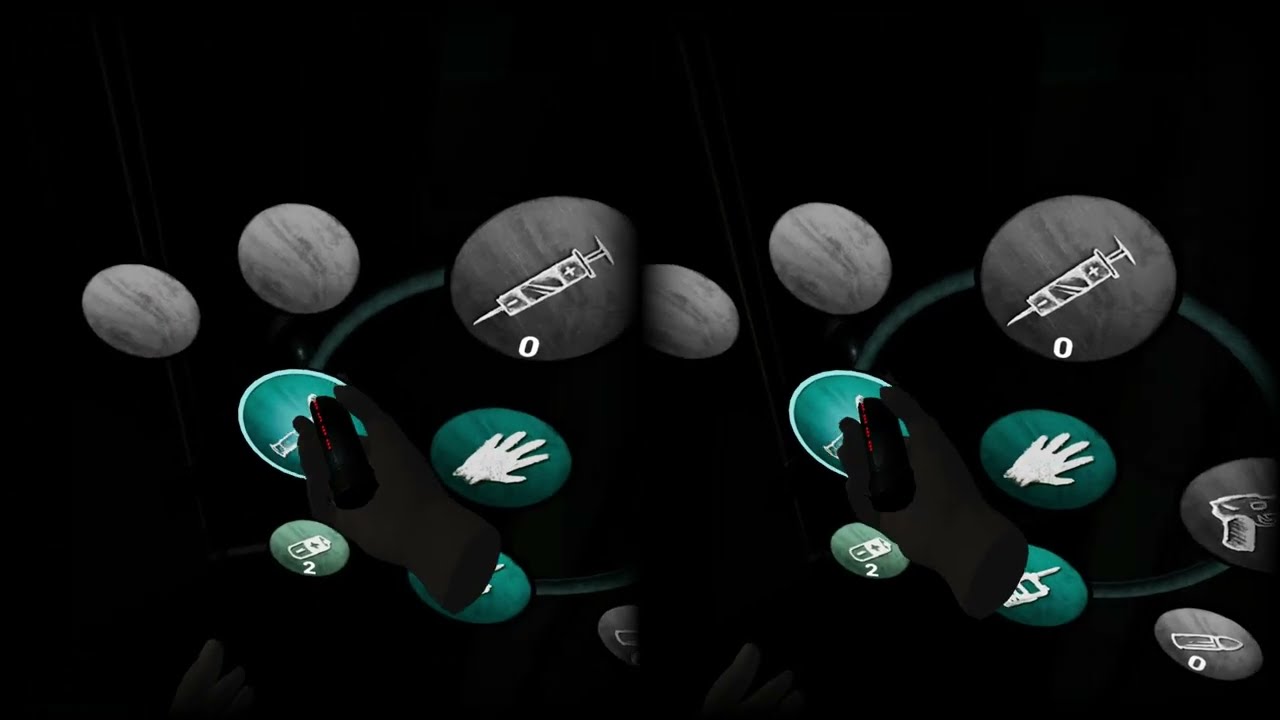The image portrays an augmented reality scene with two mirrored black-gloved hands, each holding a small black rectangular object featuring illegibly small red numbers. Dominating the center of the composition is the left hand, palm facing towards us and slightly open. Surrounding the hand is a constellation of circular disks varying in size and color, each emblazoned with distinct symbols and numbers indicative of their functions.

Near the top, within the largest circular disk positioned centrally, a syringe icon is displayed with "0" labeled beneath it, signifying the quantity held by the user. Adjacent to the thumb and index finger, another smaller green circle appears to contain a vial, though its details are partially obscured. Below the pinky, a battery icon with a "+ -" symbol and the number "2" is discernible. Centered above the wrist area lies a prominent green circle featuring a white hand symbol. Scattered around are additional grey circles with indiscernible patterns, two of which, placed near the top of the index finger, are empty or unclear in their contents.

The entire scene is set against a backdrop reminiscent of a game interface, indicating this is likely a screenshot from a virtual or augmented reality environment where these elements represent interactive or collectible items, their quantities, and statuses.